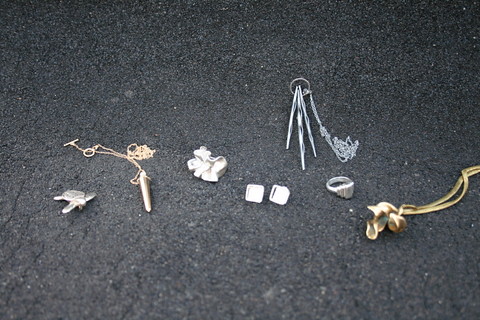The photograph captures a close-up section of a dark gray, black asphalt street showcasing various pieces of jewelry scattered across the surface. On the far left lies a pin with a flag emblazoned on it, the details of which are unclear. Near this pin, there is an intricate silver turtle brooch. Next, a striking silver necklace features three long, spike-like pendants that resemble icicles, hanging from a central ring. Adjacent to the necklace is a silver ring with a square setting. Further to the right, a delicate silver chain supports what looks like a pendant with a wadded-up ball of silver. Near this chain, two square silver earrings are positioned close together. Toward the far right side of the frame is a gold chain necklace adorned with a small gold pendant resembling bunches of petals, and one of the gold chains has a fine gold chain with a clasp, suggesting it might be a bracelet or an additional decorative element. Finally, another gold piece with some golden objects attached provides a subtle contrast to the predominantly silver display. This detailed assortment of jewelry objects, against the textured asphalt surface, gives the photo an intricate and varied visual appeal.